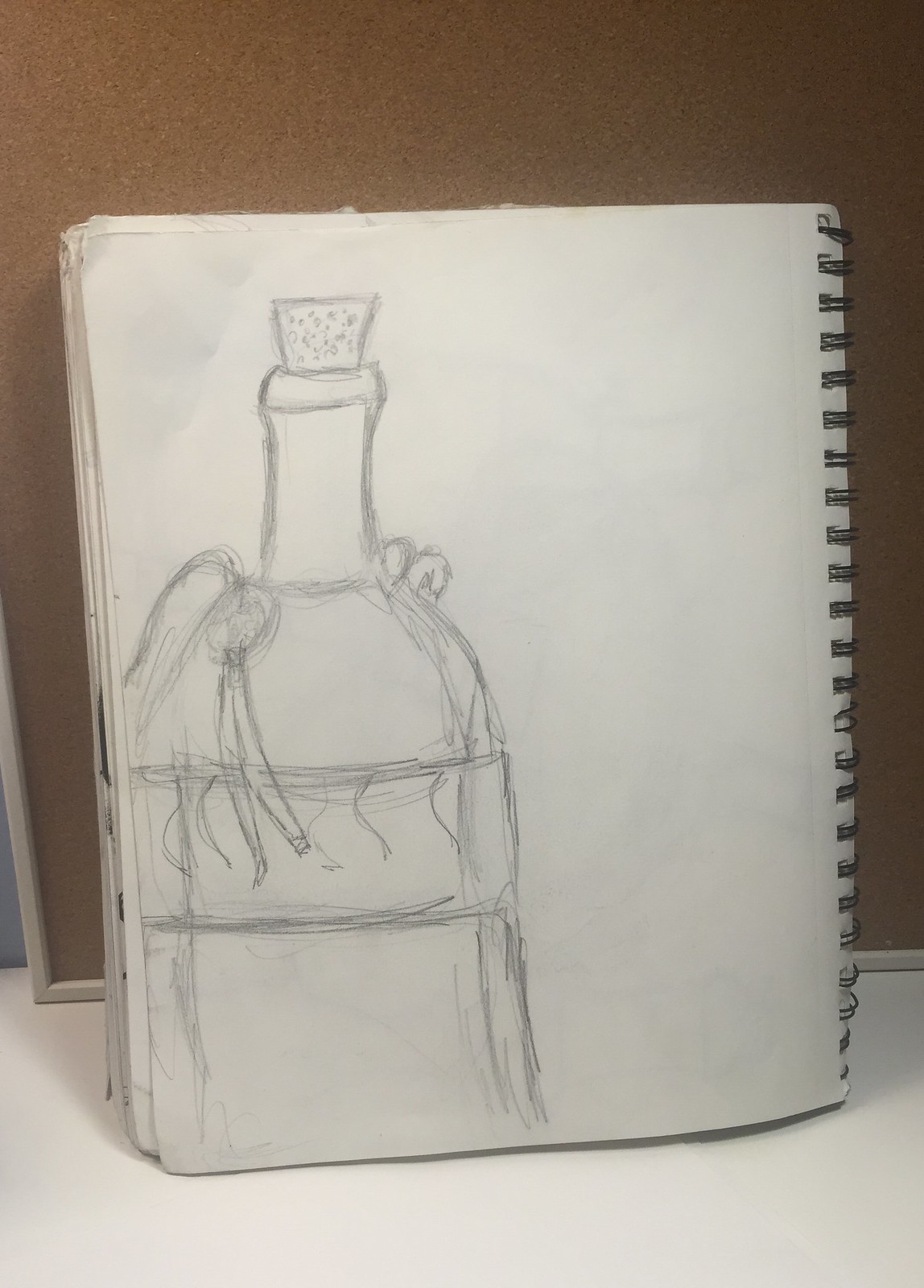In this image, a section of a brown wall borders a white countertop, accented with a thin strip of silver detailing. Resting on the countertop is a spiral-bound notebook opened to a blank, white page. On this page, a detailed pencil sketch of a large jug is prominently featured. The jug, capped with a cork at its narrow top, showcases delicate ribbons hanging from its sides. Positioned at its midsection is a label adorned with slight scribblings, contributing to its intricate design. The jug widens significantly towards its base, standing out as the focal point of the drawing. A hand, seemingly sketched in the same pencil medium, appears to be gently grasping the jug from above.